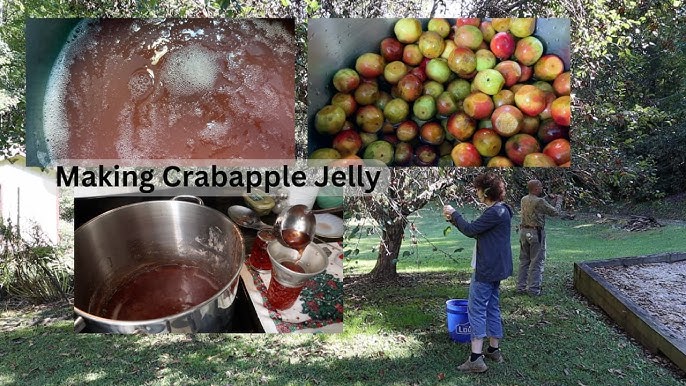The image captures a sunny daytime scene set in a lush garden, showcasing the process of making crab apple jelly. Centrally, a crab apple tree with white leaves and branches extends its reach, sheltered by the surrounding greenery. Beneath it, a woman with brown hair, dressed in a navy blue long-sleeve cardigan, blue jeans, and brown shoes, stands alongside a man in a dark green long-sleeve shirt and gray trousers. They appear to be picking crab apples from the tree, adding to the atmosphere of cultivation and harvest.

Overlaying this pastoral setting are three smaller inset images. The first depicts a pot of reddish liquid boiling, indicating the initial stages of jelly preparation. The second shows a container filled with the red and green crab apples, signifying the raw ingredients. The third image, at the bottom, features a large round stainless steel pot, with someone scooping out the finished jelly into a can, emphasizing the culmination of the cooking process.

Across the middle of the image, the title "Making Crab Apple Jelly" is prominently displayed in black text on a white background, providing context to the captured moments. To the right, a cemented or barricaded platform with soil and a sandbox-like area adds a touch of garden utility to the vibrant and detailed scene.